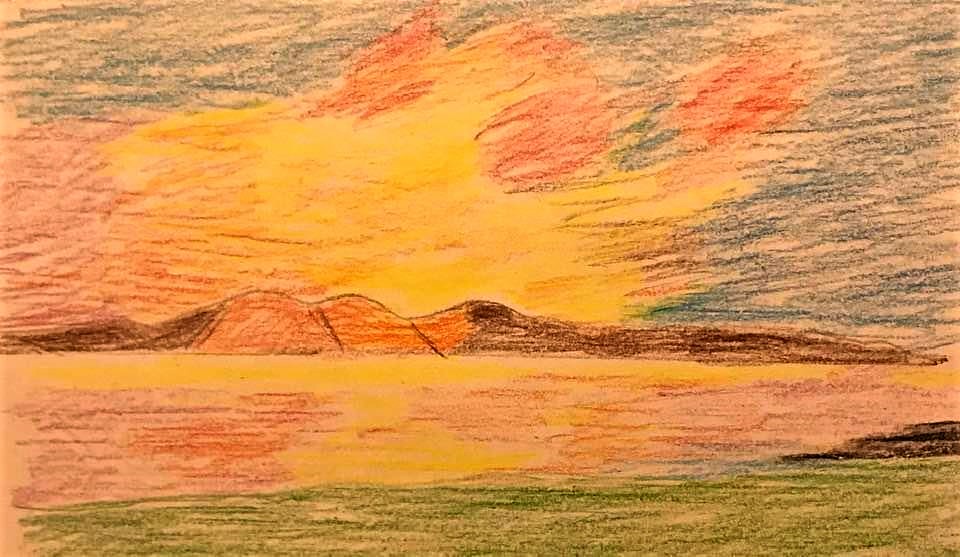The image is a hand-drawn child’s illustration, likely created with colored pencils and possibly scanned into a computer. The illustration encompasses the entire sheet of paper without any crumples or highlights. It depicts a mountainous landscape under a vibrant sky, suggesting a sunrise or sunset scene. The mountains, characterized by a series of curved humps, are primarily colored in shades of brown with tints of red.

In the foreground, there are sections of dark green and yellow with hints of olive green, resembling grass. These areas blend into the backdrop of mountains that are darker, chocolate brown on the edges and more orange in the center. 

Above the mountains, the sky is awash with a chaotic mix of colors: rich blues on the left and right, interspersed with dynamic hues of red, orange, yellow, and gold in the middle. This colorful sky likely represents the reflections of sunlight during either dawn or dusk, further emphasized by a significant yellow splotch in the middle, possibly representing the sun itself surrounded by radiating colors.

Overall, the illustration appears lively and playful, indicative of a child’s interpretation of a natural scene with an unconstrained and imaginative use of color.